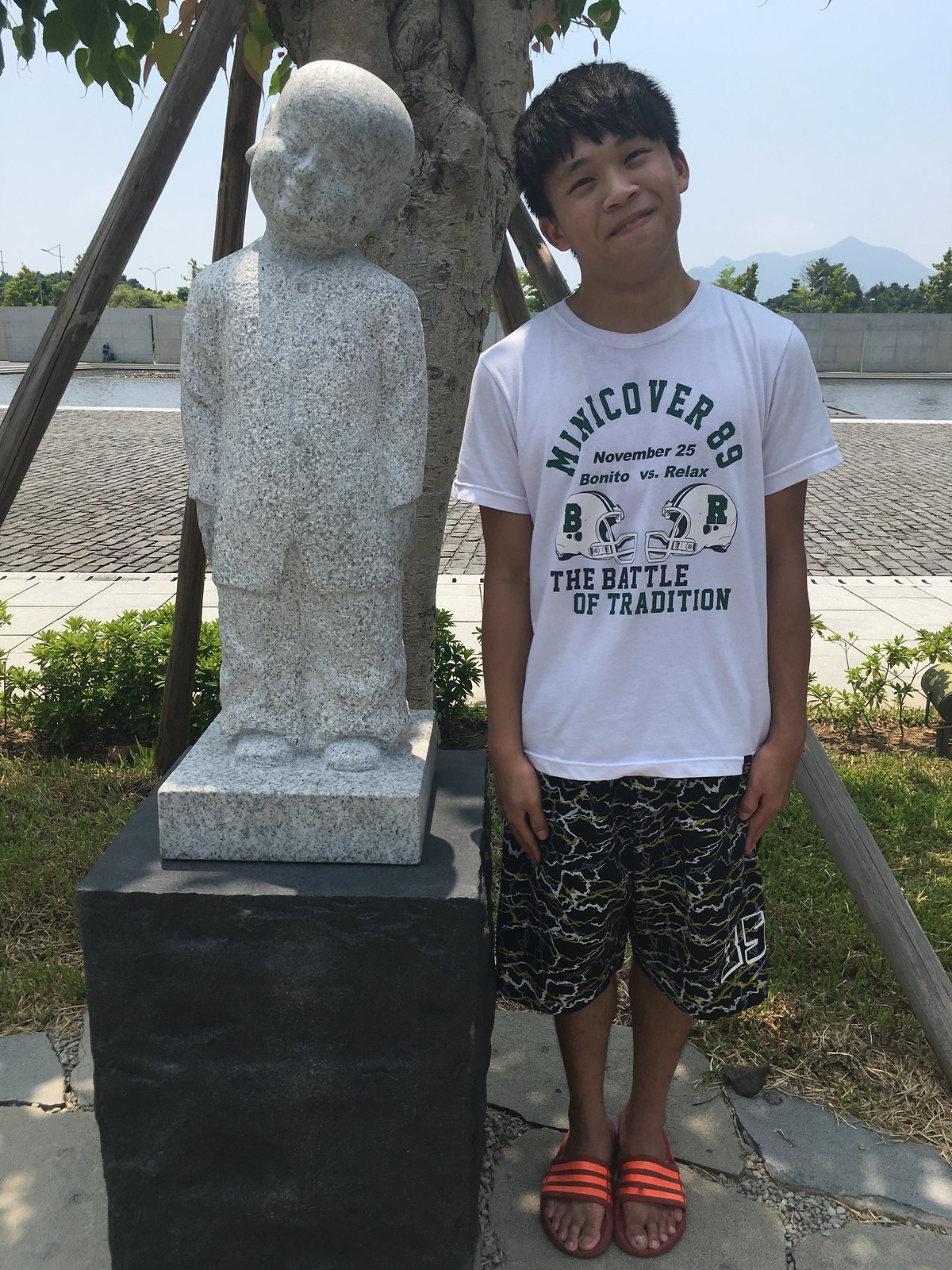In a bright, sunlit park or tourist spot, a young Asian boy stands beside a stone statue that mirrors his stance. The boy, dressed in a white t-shirt adorned with green text reading "Mini Cover 89, The Battle of Tradition" alongside two facing football helmets, and wearing dark, patterned shorts emblazoned with the number 85, gazes at the statue with his head tilted to the right. His black hair is neat, and he completes his look with red-striped sandals. The statue, perched on a black pedestal, features a young child with hands at his sides and head tilted to the left, creating a visual echo of the boy's pose. Behind them, a tree stands tall, with its trunk visible alongside some supporting pillars, casting shadows that suggest midday light. The area is alive with greenery, including ground plants and grass. Beyond the pathway that wraps around the scene, a water body glistens in the distance, bordered by a barricade wall, with a backdrop of hills rising under a clear blue sky.